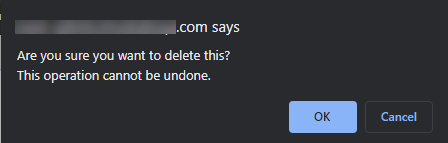This digital image features a rectangular frame with a solid black background. At the top, there is a line of text partly obscured by a gray strip, blurring out approximately two inches of information. The readable section of the text states, ".com says." Directly below that, in bold white font, the image poses the question, "Are you sure you want to delete this?" Beneath this, a warning text in the same white font reads, "This operation cannot be undone."

On the right side of the image, there are two interactive buttons. The first is a lavender-colored "OK" button, and next to it is a black "Cancel" button with lavender-colored text. The image is concluded with a polite note: "Thank you for watching."